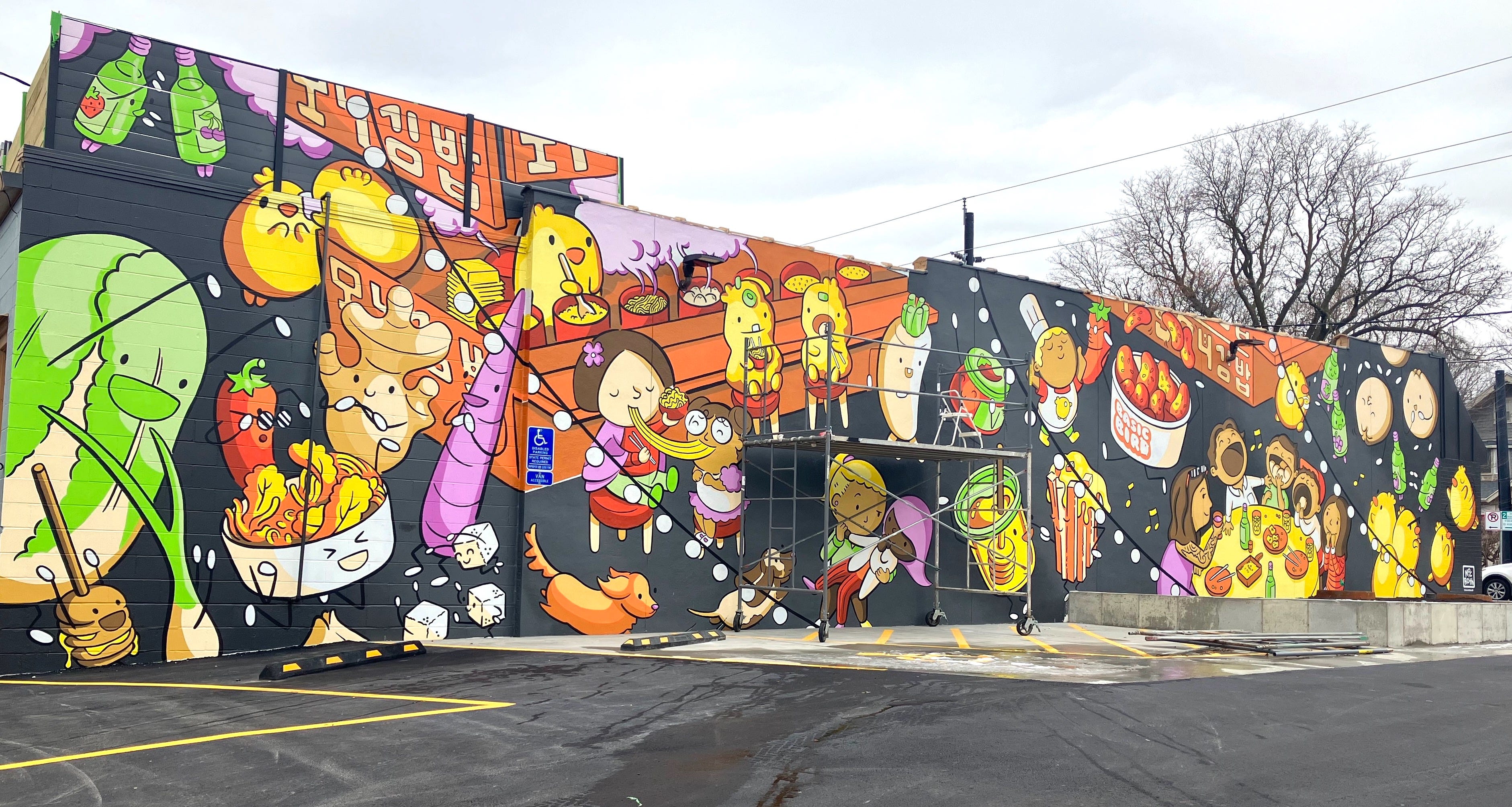We are standing in an empty parking lot that provides a perfect vantage point to view a large mural decorating the entire broadside of a black building, likely made of concrete or brick, showcasing a whimsical, anime-inspired theme. This vibrant mural, still partially under construction with visible scaffolding, is an imaginative collage of childlike drawings depicting various types of food and joyful scenes. On the left side of the mural, colorful produce like ginger, carrots, bok choy, and turnips, many with cute, anthropomorphic features like eyeballs, create a whimsical display. To the right, scenes of people enjoying food together, such as families sharing a meal and two little girls savoring spaghetti, reflect a sense of community and celebration. Scattered throughout are playful elements like meatballs on sticks, a bucket of chicken, and chickens cooking on a stove, adding to the lively and endearing charm of the mural. The overall effect is one of a vibrant, joyful art piece that brightens the urban landscape with its detailed and engaging depiction of food and camaraderie.